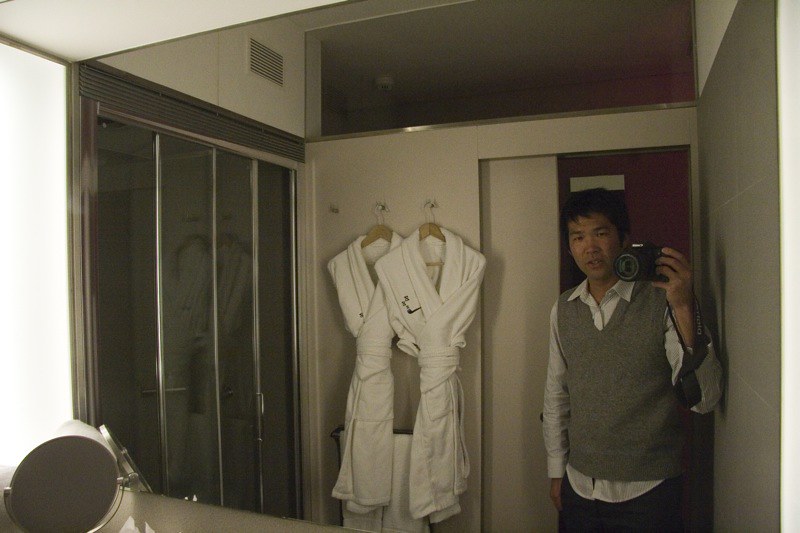This color photograph, taken indoors, shows a man of Asian descent standing in a hotel bathroom, posing for a selfie in a mirror. He has short black hair and an olive skin complexion, and he is wearing a gray v-neck sleeveless sweater vest over a long-sleeved white dress shirt, paired with black pants. He holds a black camera with white text and a long lens in his right hand. The bathroom features cream-colored walls and a dark brown door, with a pair of white bathrobes on wooden hangers above a black towel rack holding a white towel. In the reflection, the left side reveals a glass-enclosed shower, while the ceiling is flanked by white walls and a metal air vent. A countertop visible in the foreground has a metallic round item, which appears to be the back of a hairdryer.